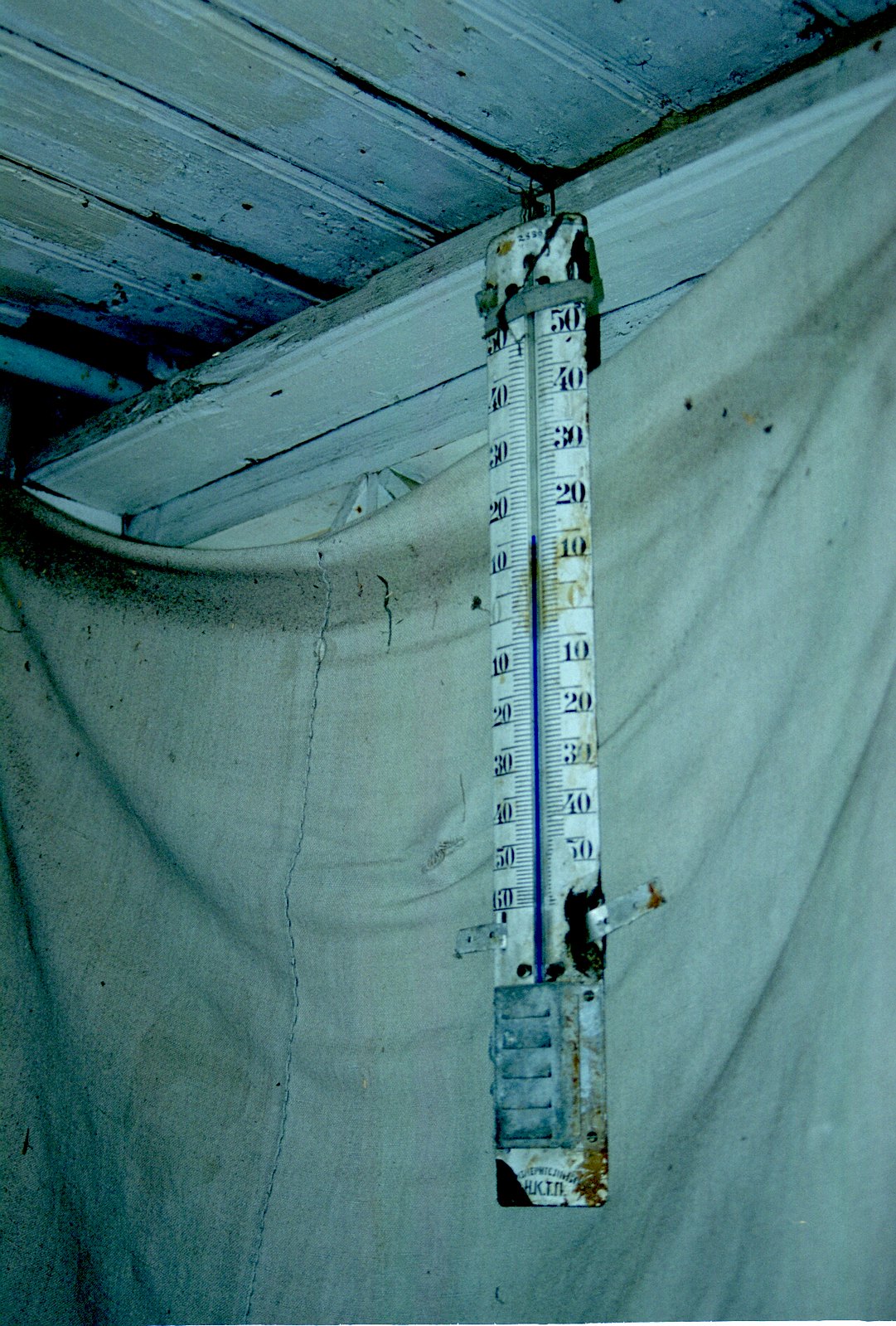This image features an old, rusted measuring tape affixed to a wall, notably deteriorated and aged. The measuring tape displays dual scales: one side progresses from 50 down to 0 and then ascends from 0 back up to 50, while a similar pattern repeats on the opposite side. Secured into the wall with screws, the tape shows significant wear, rust, and corrosion, with prominent light brown stains around the 10 and 30 marks on both scales. The wall itself is draped with a heavily stained and wrinkled blanket, further adding to the decrepit ambiance. Overhead, the wooden slats of the ceiling are also in poor condition, exhibiting signs of decay and blackened edges likely from mold or water damage. The overall scene is one of neglect and weathering, both on the measuring tape and the surrounding elements.